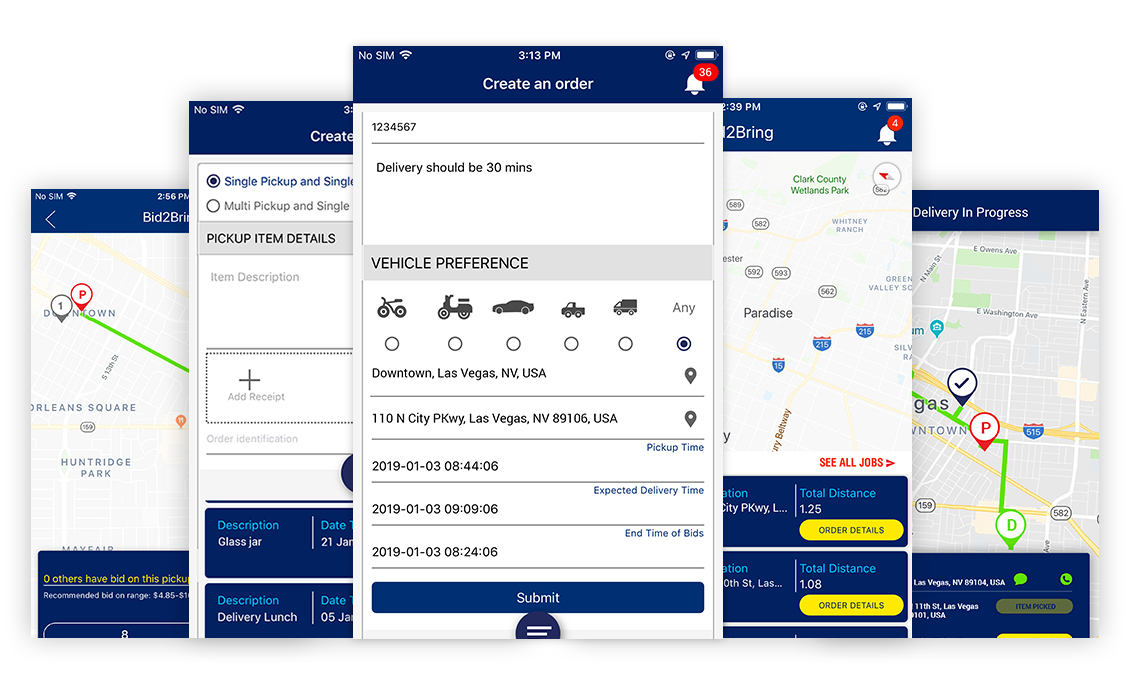The image portrays a detailed interface of what appears to be an ordering system, potentially for a service like Lowe's. At the top center of the interface, there is a prominent header that reads "Create an Order," accompanied by a blue bar displaying the current time, Wi-Fi signal strength, and a notification icon indicating multiple alerts in red.

Below the header, the primary screen displays an order summary, including an order number, and specifies that the delivery will occur within 30 minutes. The interface provides options for selecting vehicle preferences, illustrated through various vehicle emojis, with the current selection set to "Any." Additionally, it lists available pickup locations, including downtown Vegas among other options. A blue "Submit" button is prominently placed for finalizing the order.

Two other similar screens are partially visible, cascading under the main one. The first of these screens, slightly obscured, includes details about a single pickup order to the left, featuring descriptions and dates. Another screen tucked underneath maps out a potential pickup location.

On the right side, two more pop-up boxes are visible, continuing the cascading layout. These boxes offer order details for two different stores and provide information about nearby interstates and highways. Finally, to the far right of the interface, there is a map indicating the delivery location.

Overall, the image presents a complex and comprehensive ordering system interface with multiple overlapping elements for managing orders, delivery details, and pickup options.